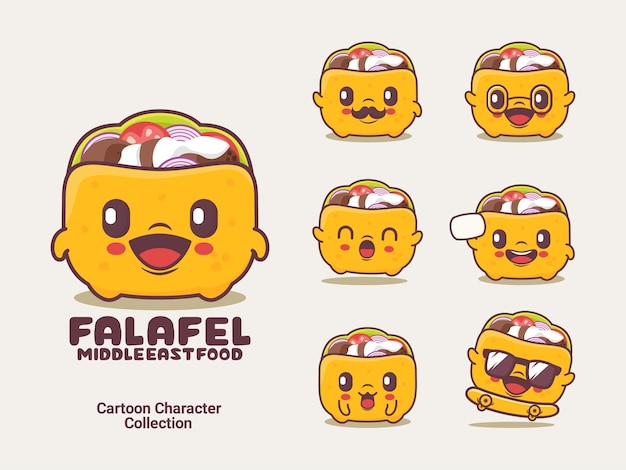The image is an advertisement for a restaurant, featuring a vibrant collection of cartoonish characters designed to promote falafel, a Middle Eastern delicacy. These adorable characters are yellow with round, red cheeks, black eyes, and open mouths revealing their little red tongues. Each character houses a meal inside, showcasing an assortment of fresh veggies.

On the right side of the image, six smaller characters are arranged in rows. Meanwhile, a larger character dominates the left side, smiling with an open mouth. Beneath this larger character, the text reads: "Falafel, Middle Eastern Food" and "Cartoon Character Collection."

The diverse array of characters includes one sporting a little black mustache with a smile, one wearing glasses, another energetically hopping up and down with closed eyes, and one holding a small white object in its hand. Additionally, there is a character resembling a dog, complete with floppy ears and a tongue hanging out, along with another cool character riding a skateboard and wearing sunglasses. This colorful and playful ensemble invites viewers to enjoy a fun and tasty dining experience.